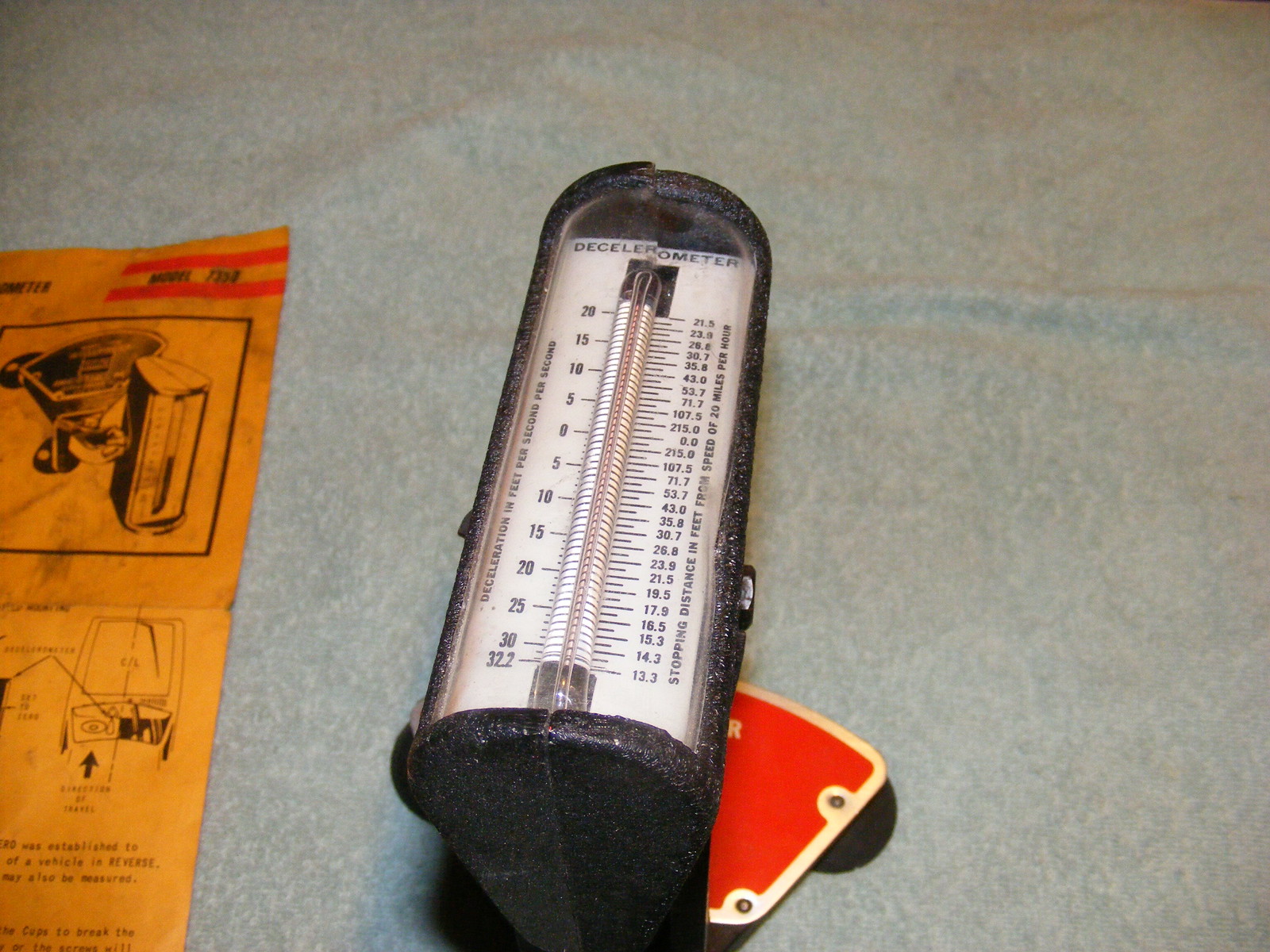A low-quality 720p landscape image set against a slightly wrinkled gray sheet backdrop. On the left edge, there's a partially visible orange sticker or label, featuring black illustrations and instructions related to a wheelbarrow and a water heater. The main focus is an oval-shaped decelerometer, outlined in a black marbled texture. The face of the decelerometer is white with the word "Decelerometer" in black at the top. It displays two sets of black numbers: the left side ranges from 0 to 20, and the right side ranges from 0.0 to 21.5, then down to 13.3. At the center, there's a thermometer-style gauge with a red background, indicating measurement markings.